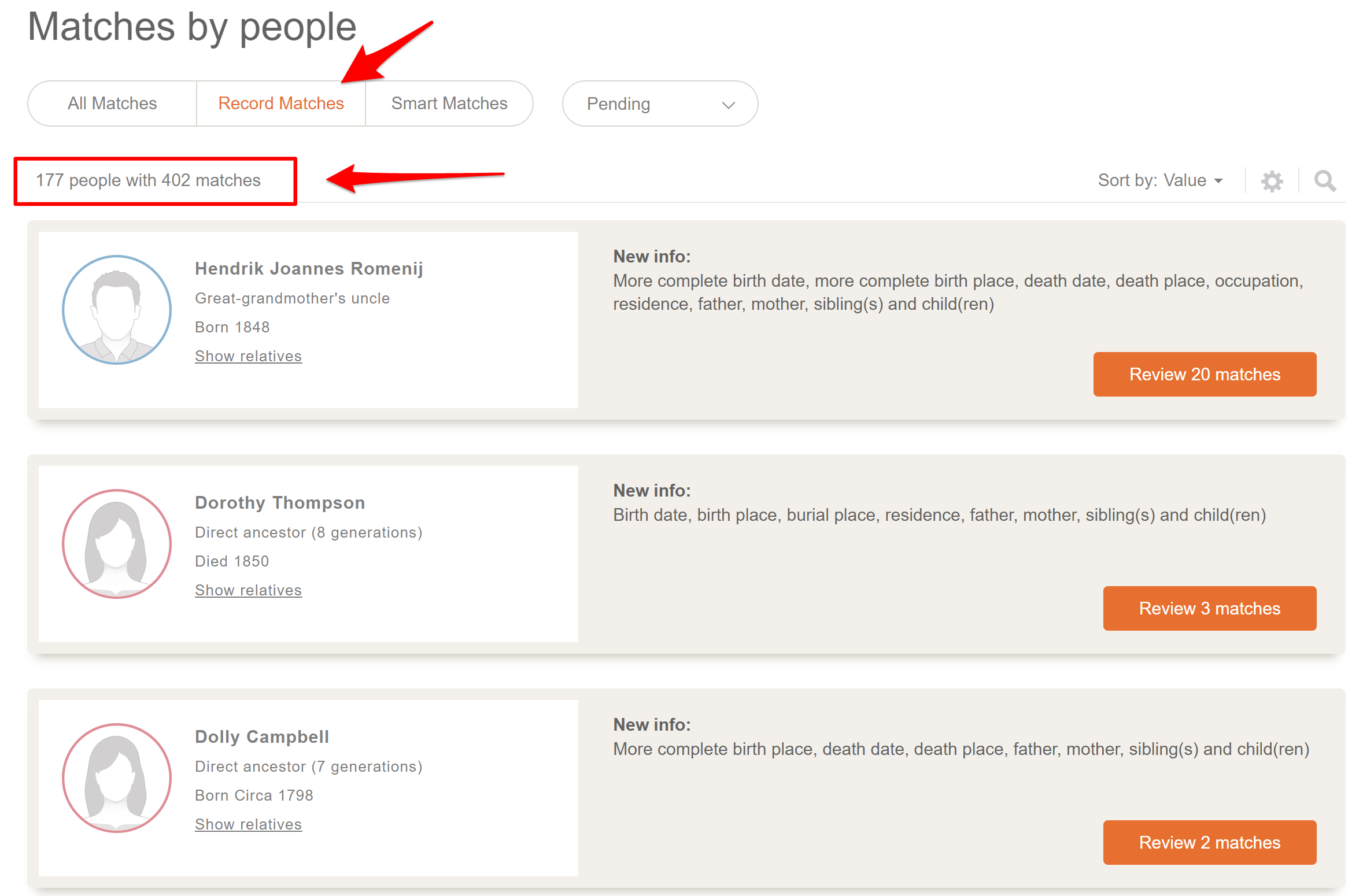This is a cropped screenshot from an unidentified genealogical website, displaying various match categories and results. At the top, navigational tabs labeled "Matches by People," "All Matches," "Record Matches," "Smart Matches," and "Pending" are visible, with "Record Matches" being highlighted by a red arrow and selected. Below, there's a section titled "177 People with 402 Matches," heavily emphasized with a red outline and an arrow pointing from the right.

In the main part of the screenshot, information about specific ancestors is listed. One highlighted individual is Hendrick Joannes Romenig, identified as a great grandmother's uncle, born in 1848. Metadata fields related to him include a more complete birth date and birthplace, death date, death place, occupation, residence, father, mother, siblings, and children. Users are prompted to "Review 20 Matches."

Another entry highlights Dorothy Thompson, a direct ancestor from eight generations back who died in 1850. Additional fields include birth date, birthplace, burial place, residence, father, mother, siblings, and children with a call to "Review 3 Matches."

Lastly, Dolly Campbell, a direct ancestor from seven generations back born circa 1798, is noted. Her profile contains more complete birthplace, death date, death place, father, mother, siblings, and children information. Users are invited to "Review 2 Matches."

Overall, the screenshot details the functionality and information provided by the genealogy website, focusing on advanced family history data and user interaction options for reviewing matches.